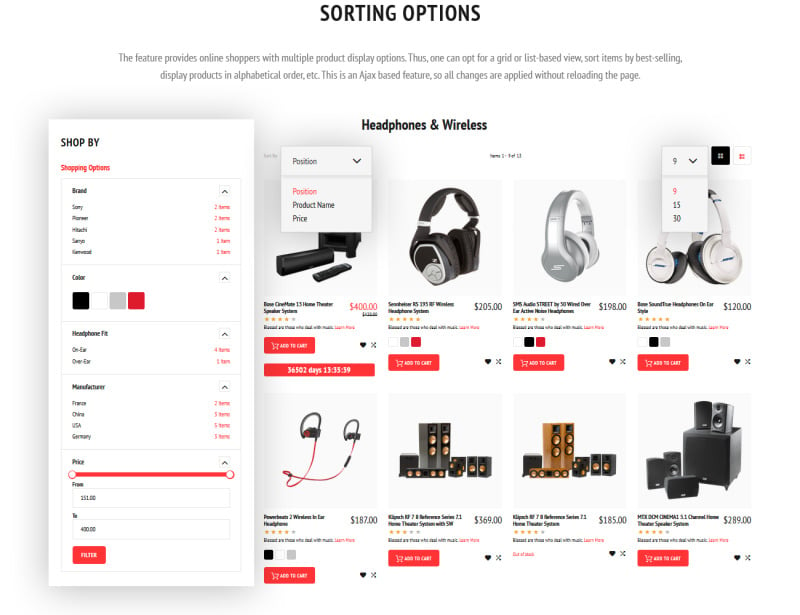The image showcases a web shopping interface focused on the sale of headphones. At the very top, in large bold letters, it reads "Sorting Options," with additional explanatory text underneath in smaller gray font. This feature allows online shoppers to choose between different product display configurations, such as a grid or list layout. Users can sort items based on various criteria like best selling or alphabetical order. The sorting functionality is AJAX-based, enabling real-time updates without requiring the page to reload.

In this particular example, the webpage is a demo, indicated by the heading "Headphones and Wireless" at the top. Below this heading, there is a 4 by 2 grid displaying a variety of headphone models. At the top of the display area, there are additional sorting options, including one labeled "Position," which appears to filter the products based on their names in a machine-generated alphabetical order.